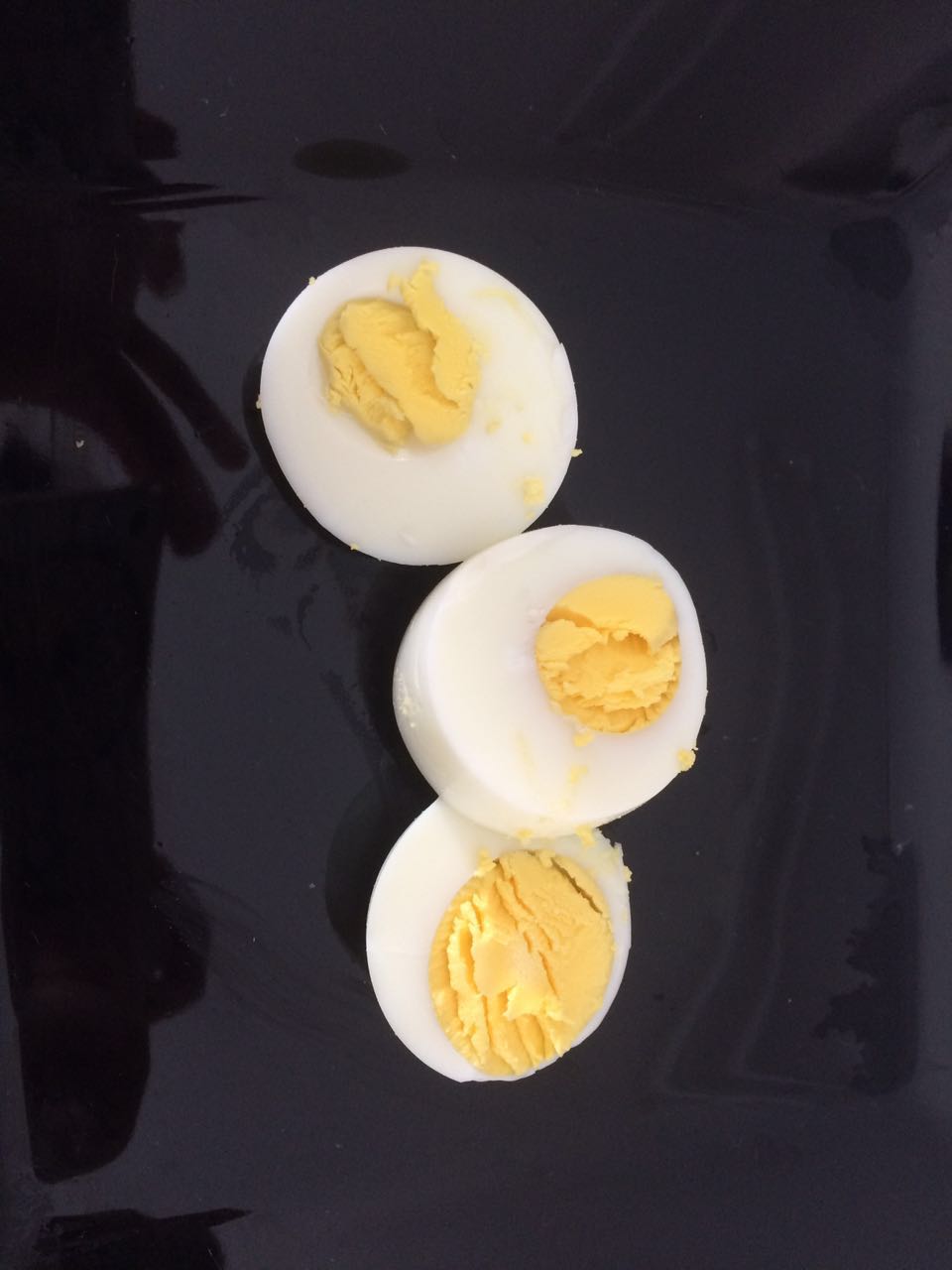In this photograph, three slices of hard-boiled egg are arranged in a vertical line against a highly reflective, black background. The background almost resembles the glossy surface of a car hood due to its smooth, shiny, and reflective texture, which captures abstract shapes. Each egg slice reveals distinct details: the top slice shows the yolk slightly smeared onto the white, with only a small portion exposed. The middle slice has a more centered yolk, offering a deeper look yet still minimal in size. The bottom slice features the largest yolk section, protruding significantly more than the others. The yolks are a vibrant yellow, contrasting sharply with the pristine white of the egg whites, highlighting the simple yet striking composition of the image.